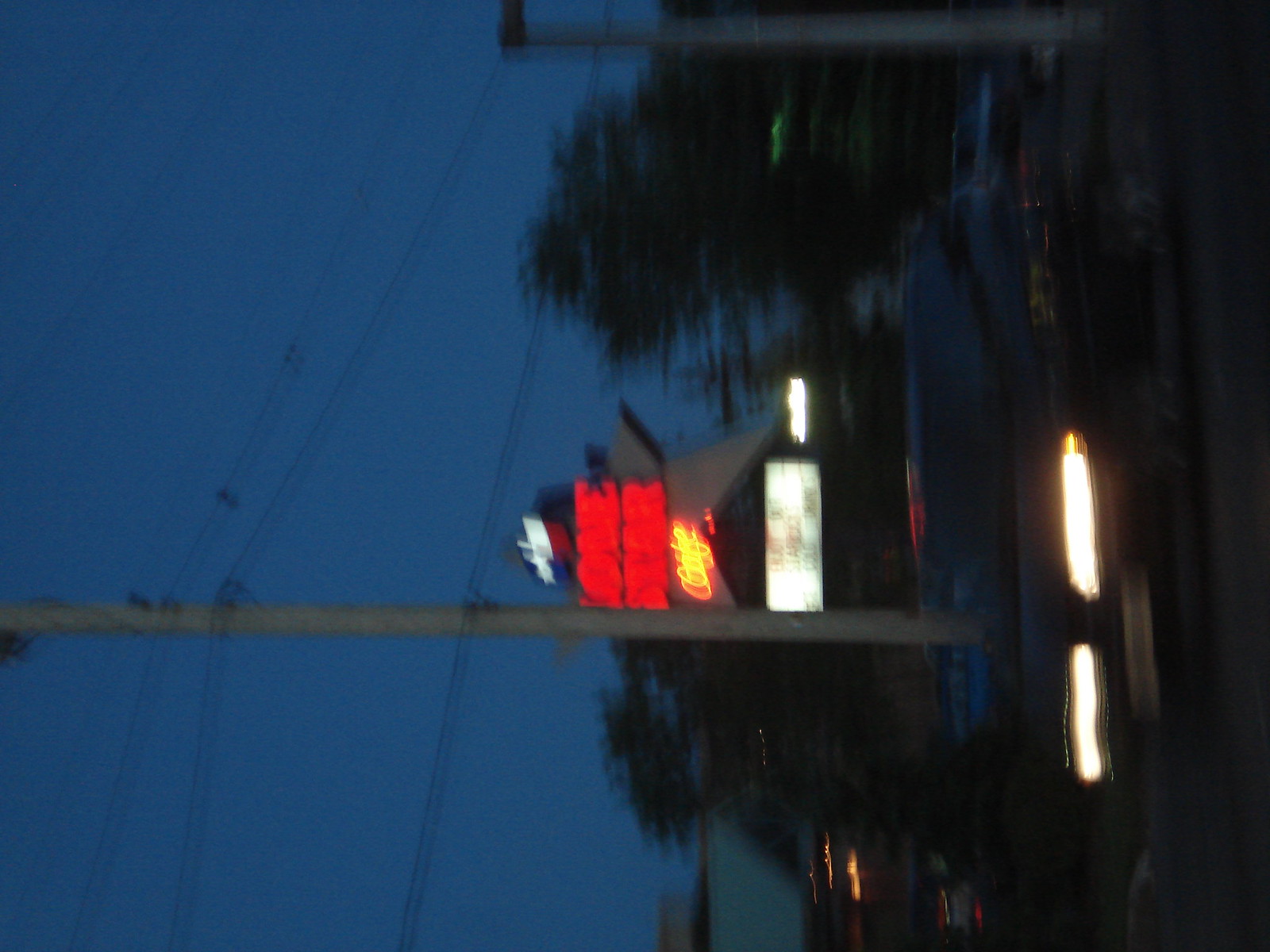This detailed night-time colour photograph, currently oriented in landscape but intended to be viewed in portrait (rotated 90 degrees clockwise), captures a scene featuring a long-exposure blur of a vehicle. The vehicle, driving diagonally from the right towards the lower left, boasts elongated and undulating illuminated headlights due to the motion blur. On the left side of the image, a telegraph pole stretches upwards with wires extending horizontally in both directions, anchoring the scene. Just to the right of this pole, an illuminated sign reads "Lone Star" in red, suggesting the location might be in Texas, USA. Below the "Lone Star" sign, partially obscured by motion blur, is a yellow-lit sign reading "Café," indicating the presence of the Lone Star Café. Behind the telegraph pole and these signs, the establishment’s façade showcases a red and yellow color scheme, with a grey star-shaped logo incorporating a cup design. Additionally, a black vehicle with its headlights on is positioned towards the right side, while the dark bluish sky and trees frame the scene.